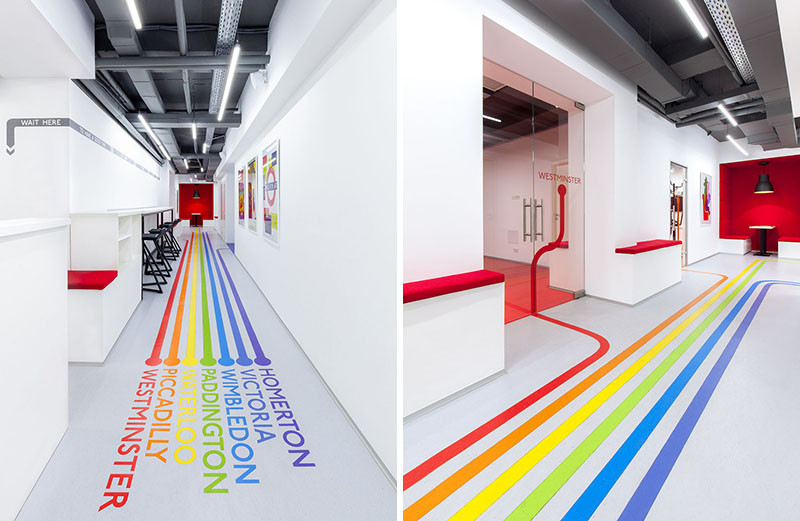The image depicts two photographs of the same narrow indoor hallway taken from different angles within a business or public area. The hallway, characterized by its white floor adorned with colorful lines and matching text, features stripes in red, orange, yellow, green, blue, and purple that guide towards different directions. Each stripe has corresponding text, such as "Homerton" for purple, "Victoria" for blue, "Wimbledon" for light blue, "Paddington" for green, "Waterloo" for yellow, "Piccadilly" for orange, and "Westminster" for red. The walls of the hallway are white, decorated intermittently with posters, and the roof is gray, illuminated by tube lights emitting white light. The hallway concludes at a striking red front wall, adding a bold element to the otherwise muted color scheme. The setup suggests a navigational purpose, potentially leading to various English locales, hinting at a connection to a transit or train station.